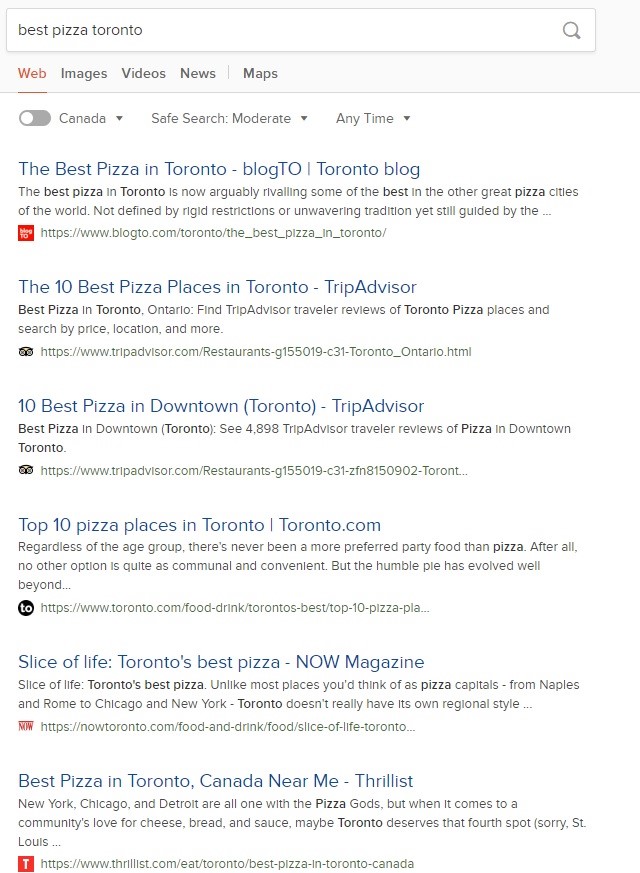**Screenshot Description: Detailed Overview of Search Results for "Best Pizza in Toronto"**

In this screenshot, we see the results page for a Google search query "best pizza in Toronto." Starting from the top, the search bar prominently displays the query, while below it are various search categories: Web, Images, Videos, News, and Maps, with the Web section highlighted in red, indicating it's the current active tab.

Just beneath these categories, a few filter options can be seen: a location filter set to Canada, a SafeSearch filter set to Moderate, and a time filter set to Any Time.

Following this, the main search results appear as a list. The first result is from blogTO, titled "The Best Pizza in Toronto." The snippet from this article suggests that Toronto's pizza rivals some of the best in other great pizza cities, remaining unrestricted by traditional norms yet still guided by foundational elements, and includes a link to the full article.

The second result is from TripAdvisor, titled "10 Best Places in Toronto" with the subtitle "Best pizza in Toronto, Ontario." It mentions that the list is based on TripAdvisor travel reviews, categorized by price, location, and more, with an associated link.

The third result, also from TripAdvisor, is titled "10 Best Pizza in Downtown Toronto" and includes review code C4898. It similarly highlights traveler reviews for the best pizza places specifically in downtown Toronto, with another link provided.

The fourth result comes from Toronto.com, titled "10 Best Pizza Places in Toronto." The excerpt notes pizza's popularity as a communal and convenient party food and alludes to the evolution of the pizza with another link included.

The fifth listing is from NOW Magazine, titled "Slice of Life: Toronto's Best Pizza." It compares Toronto's pizza scene to other famous pizza capitals like Naples, Rome, Chicago, and New York, pointing out that Toronto lacks a distinct regional style. A link to this article is also present.

Finally, the sixth result is from Thrillist, titled "Best Pizza in Toronto, Canada Near Me." This snippet mentions Toronto as potentially being the fourth-best city for pizza, rivaling New York, Chicago, and Detroit, and humorously apologizes to St. Louis. A link to Thrillist’s article is provided at the end.

The overall scene of the screenshot gives a structured view of diverse sources, all offering insights into where to find the best pizza in Toronto.